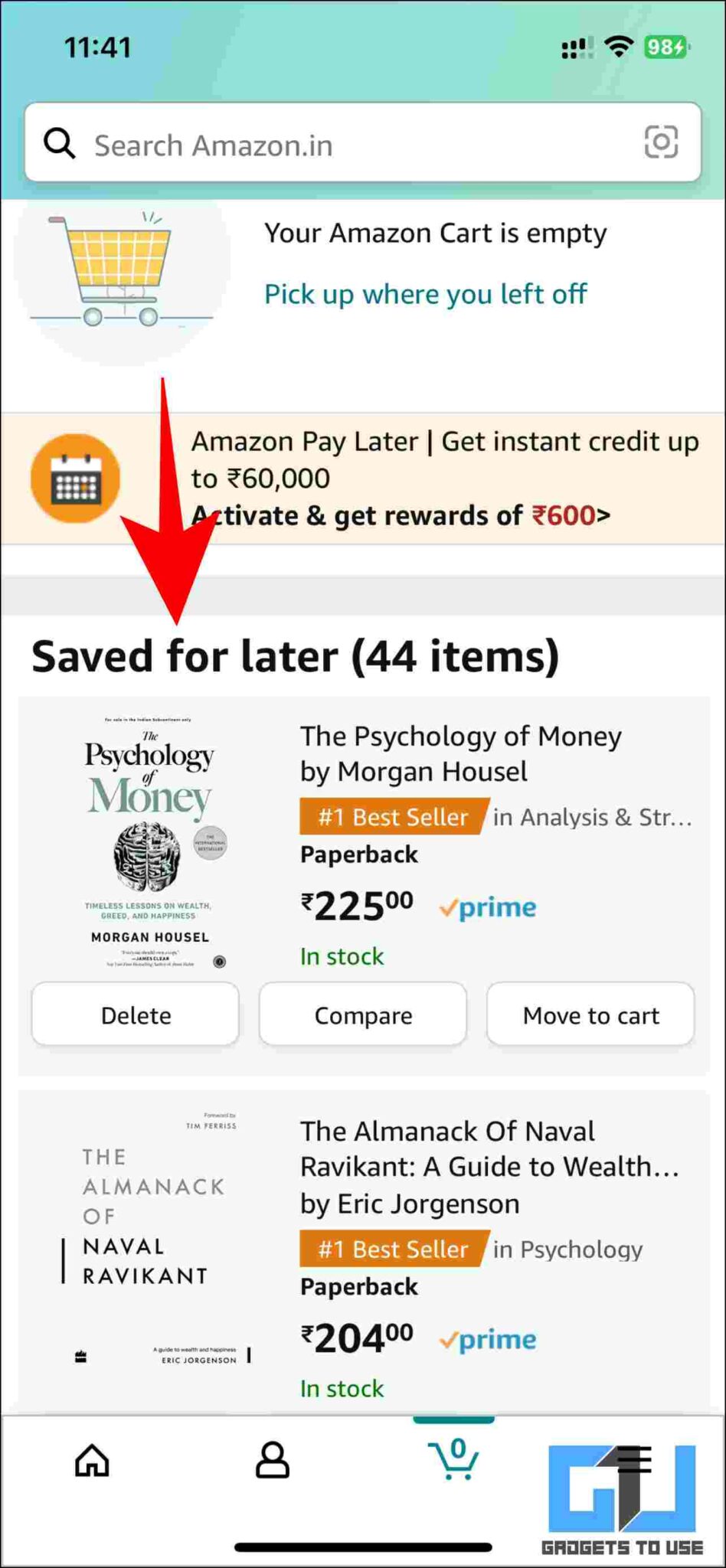The image displays a shopping platform on a smartphone screen with the following details:

- **Top Section**: 
  - **Time**: 11:41 AM displayed in the top left corner.
  - **Icons**: Wi-Fi icon and a 98% battery indicator in the top right corner.
  - **Search Bar**: Positioned just below the icons, featuring a white background.

- **Shopping Website Overview**:
  - **Top Area**: 
    - A gray circle containing an orange shopping cart icon.
    - Adjacent text reads, "Your Amazon cart is empty."
    - Blue text below that states, "Pick up where you left off."
  - **Promotional Banner**: 
    - Pink background with the text, "Amazon Pay Later."
    - Promotes "Get instant credit up to $60,000" and "Activate and get rewards of $600 plus" in red text.
    - Features an orange calendar icon to the left of the promotional text.
  
- **Saved for Later Section**: 
  - Displays the text, "Saved for later (44 items)" in black text on a white background.
  - Below this line, the background transitions to light gray.

- **Product Listings**:
  - **First Product**: 
    - "The Psychology of Money" by Morgan Housel.
    - Marked as a "#1 Bestseller," available in paperback for $225 (currency not specified).
    - Includes options: "Delete," "Compare," and "Move to Cart," all in black text on a white background.
  - **Second Product**: 
    - "The Almanac of Naval Ravikant: A Guide to Wealth" by Eric Jorgensen.
    - Also a "#1 Bestseller," priced at $204.
  - Both items are noted as in stock.

- **Bottom Navigation Menu**: 
  - Icons for Home, Profile, Shopping Cart, all on a white background.